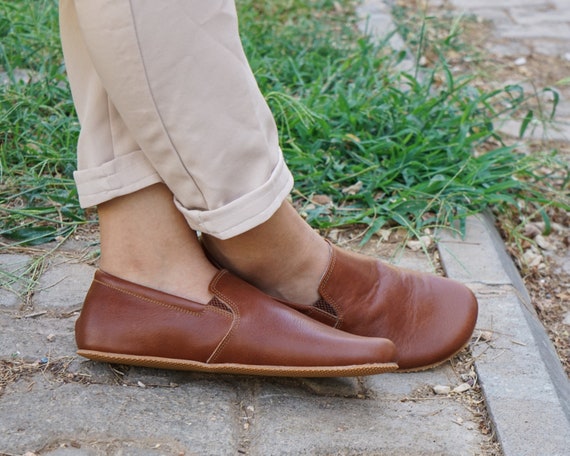This color photograph captures a detailed view of someone's lower legs from approximately the mid-shin down. The individual, who has light brown skin, or possibly Caucasian, is wearing khaki pants that are rolled and cuffed up to the ankles. Their brown leather loafers, featuring a light brown lining at the bottom, rest on a gray paved sidewalk. The right foot is slightly crossed over the left, suggesting a relaxed stance likely leaning against something for balance. Surrounding the sidewalk is lush, long green grass interspersed with patches of dried vegetation and dandelion weeds. Small pebbles are visible in the foreground, adding a touch of texture to the scene. There are no other people, animals, or identifiable logos in the photograph.